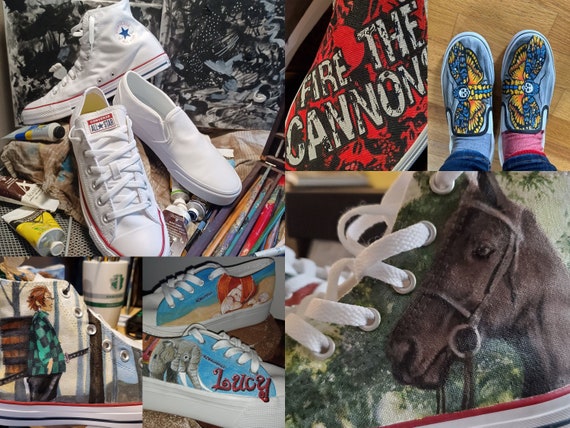This image is a detailed collage featuring painted shoes and art supplies. In the top left corner, there's a pair of classic white Chuck Taylors with a blue star on the tongue, labeled "All Star," and the Converse logo in red. Surrounding the shoes are various coloring pencils and paint supplies. Below this, a shoe displays an illustration of a person with a sword in the woods, depicted on a green background that resembles trees. To its right, a pair of white and blue shoes shows a red-headed woman above the word "Lucy" alongside an elephant. In the top right corner, a blue shoe is adorned with moths and the phrase "Fire the Cannon." The bottom right features a close-up shot of a green shoe with white laces and a painted brown horse with a bridle looking to the left. All these artistic designs showcase the use of colorful paint tubes and brushes, emphasizing the theme of creative customization of footwear.